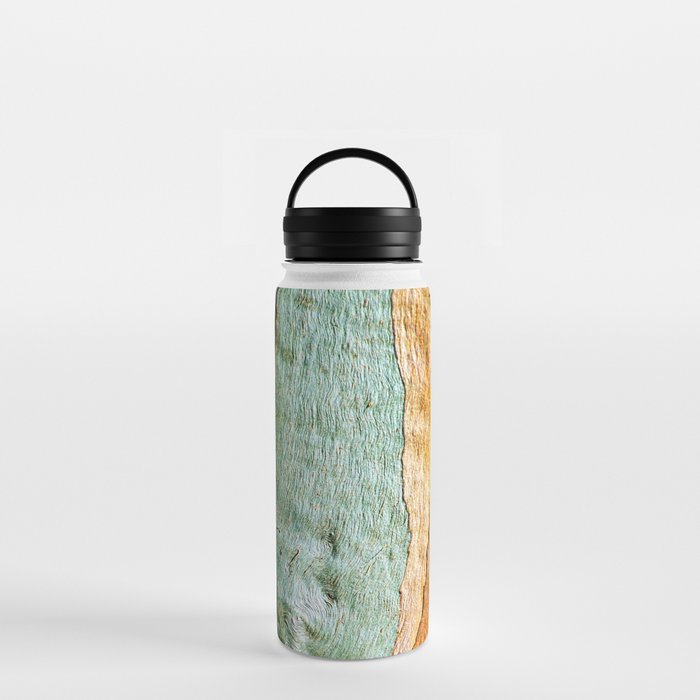This image depicts a tall, cylindrical water thermos with a sleek, modern design. The body of the thermos is predominantly wrapped in an artistic, textured material that mimics the grain of wood, combining a distressed light green area on the left and a brownish tan section on the right. The pattern appears to be made of some kind of crumpled paper, giving it a handmade, rustic appearance. The thermos features a classic black screw-on top made of plastic, complete with a convenient semi-circular handle for easy carrying. The whole setup rests on a clean, white surface against a plain off-white background.